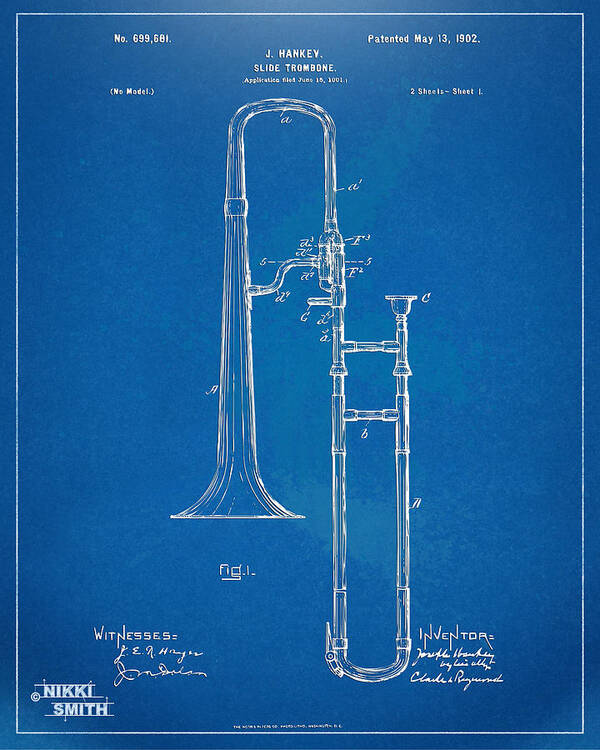This image showcases a patent blueprint for a slide trombone against a dark blue background, with intricate white line details. Centrally featured is the trombone design with its mouthpiece on the far right, extending upward, and the tubing curving downwards, leftward, upward again, and finally leftward and downward to form a complete outline. The blueprint includes meticulous labels: "patented May 13, 1902" appears on the top right, while "no. 699681" is displayed on the top left, both in a typewriter-like font. Above the trombone's upper arch, "J. Hanke, slide trombone" is prominently noted, with the application date of "1st June 15, 1901" immediately below. "No model" is inscribed to the bottom left, and within parentheses to the right, it states "two sheets, sheet one." Near the trombone's output opening, the term "fig 1" is noted, with the G's lower loop extending leftwards. On the bottom right, beside "inventor," appear two cursive signatures of the inventors, Jonathan Hanke and Charles Raymond. Witnesses' endorsements are hand-signed on the left in cursive, accompanied by the name "Nikki Smith" in bold on the bottom left. This detailed visual, resembling a slide trombone's architectural schematic, is a historical testament to its patented design.